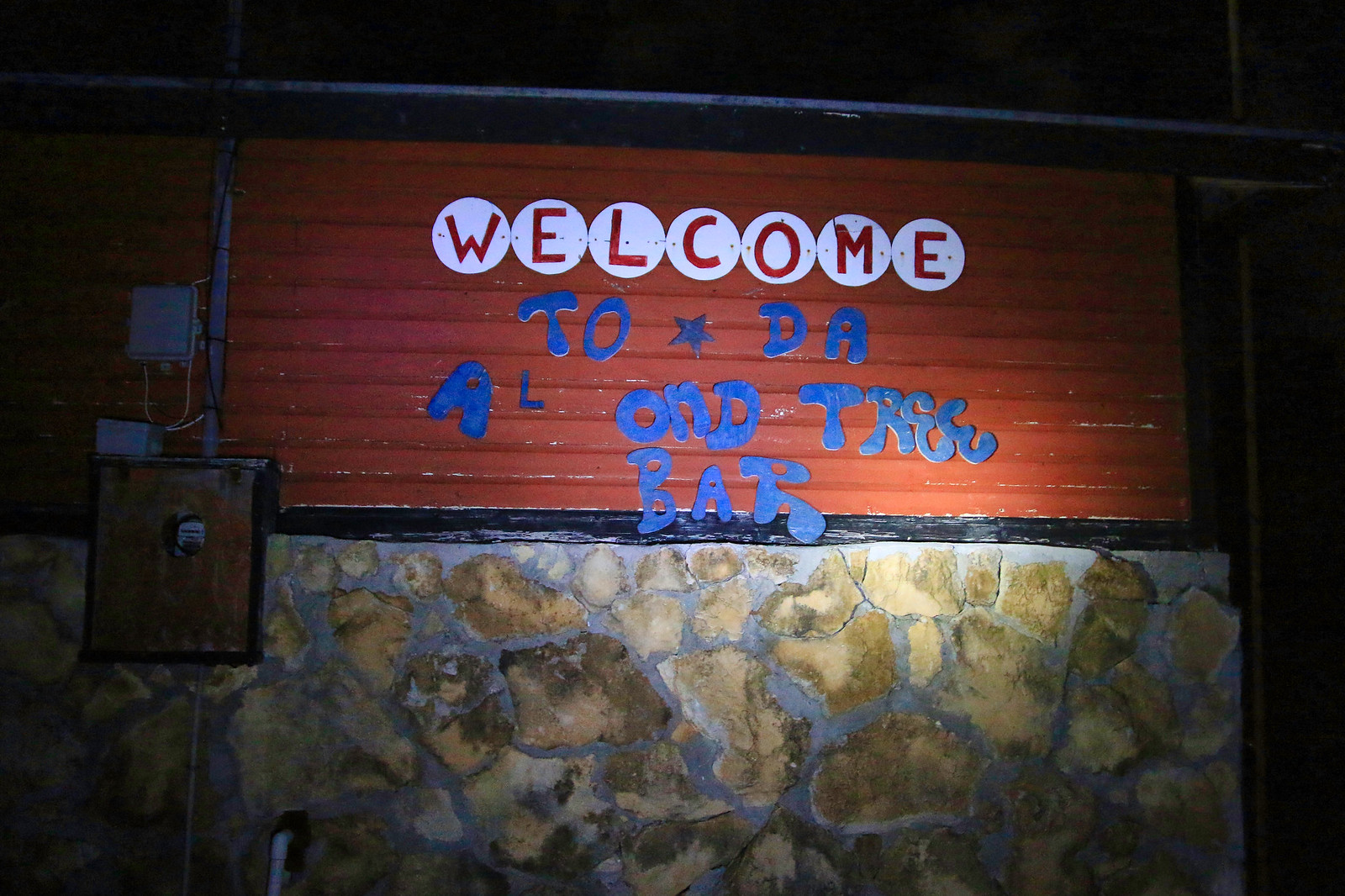This nighttime image features a roughly constructed stone wall, characterized by cracked and yellowed tan and brownish stones held together with sloppy gray cement grout. A black stripe sits atop the stone wall, followed by red, horizontally laid wooden boards. Above these boards are multiple white circles containing red or orange letters that spell out "WELCOME." Beneath these circles, in cartoonish blue block letters, it seemingly reads "TO DA ALL ON TREE BAR," though several letters appear to be missing or have fallen off. The scene appears to be illuminated by artificial light, perhaps from a flashlight or car headlights. To the left of the sign, there is a rusted metal box with a pole rising above it, accompanied by smaller white and gray boxes and pipes, adding to the derelict feel of the setting.